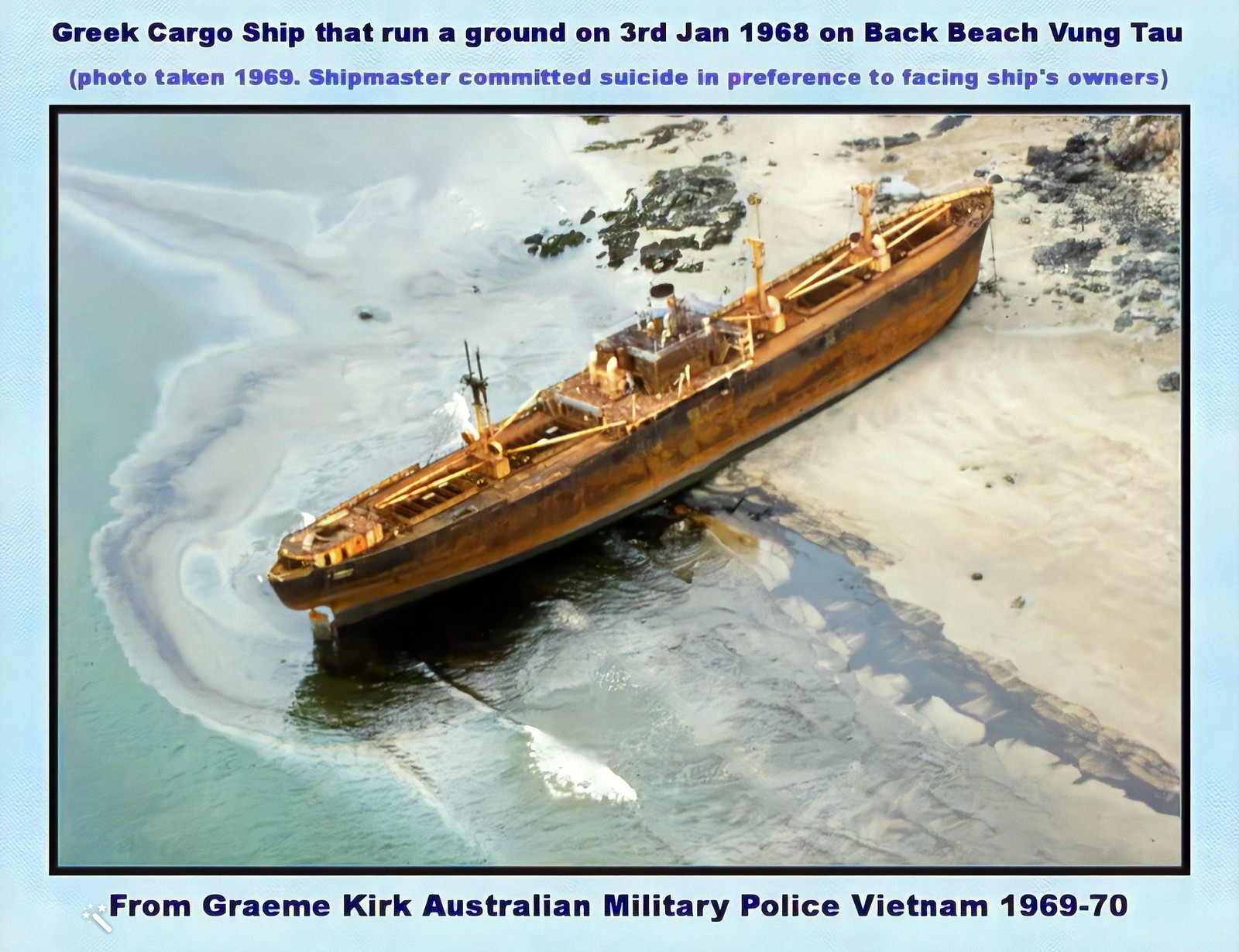The image is a color photograph of an old Greek cargo ship that ran aground on Back Beach, Vung Tau, Vietnam on January 3, 1968. The picture, taken in 1969 by Graham Kirk of the Australian Military Police, Vietnam, showcases the abandoned vessel partly submerged in turquoise water with the bow or stern resting on the brown sand and rocky shoreline. A blue border surrounds the photograph with black header text that reads: "Greek cargo ship that run aground on 3rd January 1968 on Back Beach, Vung Tau." Beneath the photograph, it notes in blue text: "Photo taken 1969. Ship master committed suicide in preference to facing the ship's owners." The rust-red ship appears to be leaking black oil into the water, adding to the scene's desolation and historical poignancy.